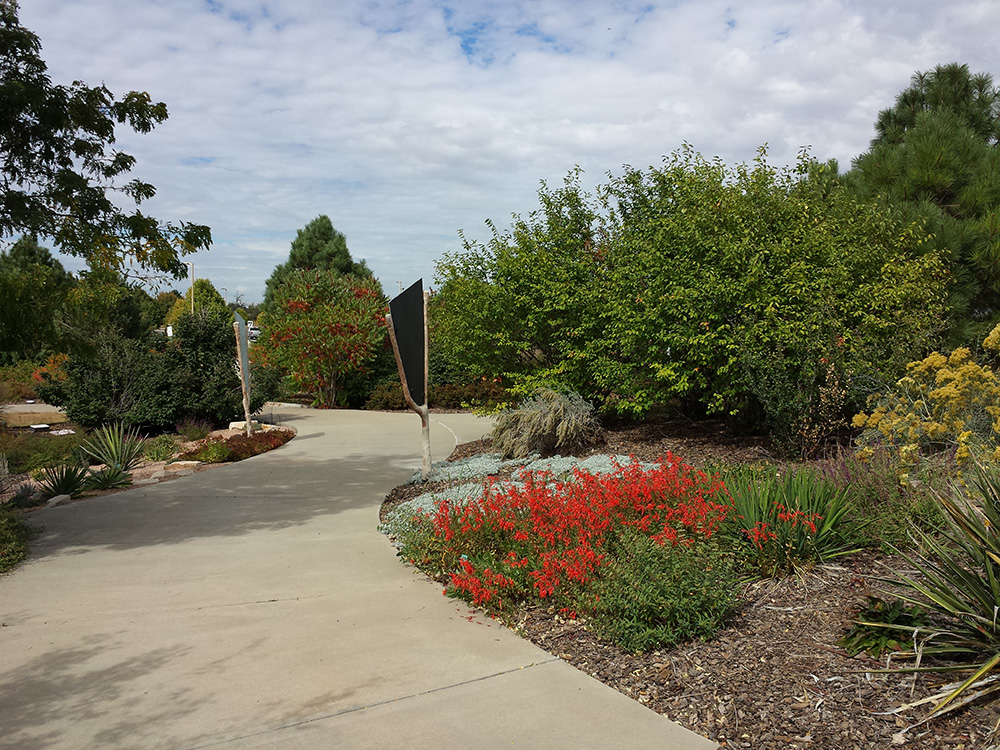The image captures a lush, manicured garden area that resembles a well-maintained park or arboretum. At the center, there's a wide concrete pathway lined with various plants and trees. On the right side of the path, you can see a striking arrangement of flora: a low-growing red flowering plant, followed by a yellow plant, some aloe vera, tall plain green bushes, and a bush with red leaves further back. There’s also a black flag on a wooden post. On the left side, spiky plants emerge from a rock border along with a noticeable bush, and in the distance, a part of a tall tree is visible. Near the left side of the path, there's a white wooden post with more mulch and flower beds. Both sides of the pathway feature brown mulch beds interspersed with low plants, long grasses, and red and yellow blooms. The sky is blue but partially overcast with numerous clouds, giving a somewhat cloudy ambiance. In the far background, glimpses of small white buildings or houses can be seen. Overall, the scene conveys a tranquil daytime setting with a mix of vibrant plant life and thoughtful landscaping.